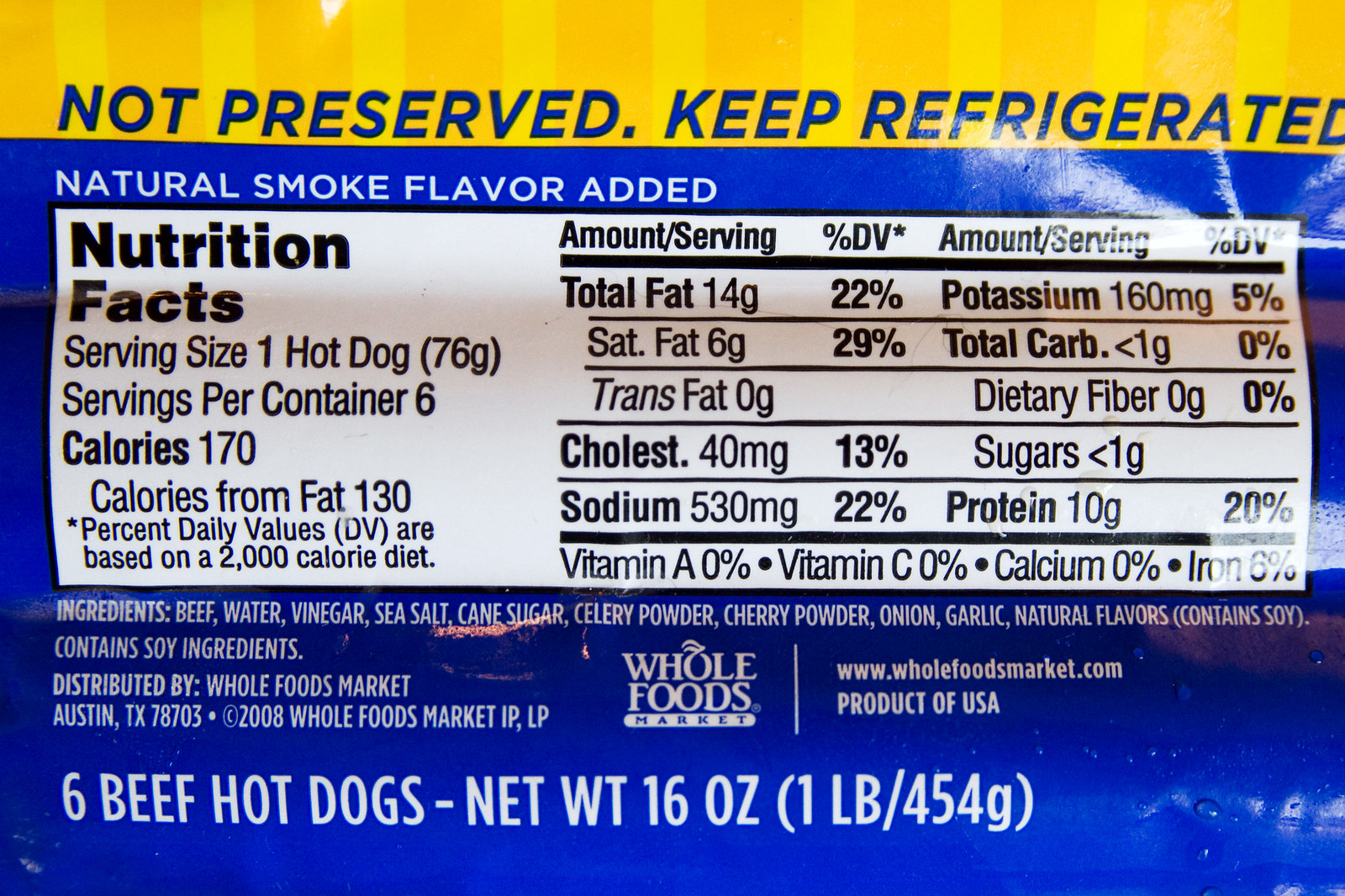This is a color photograph of a food package, prominently displaying the Nutrition Facts label at the top of the image. The package features yellow and orange stripes, above which is the message "Not Preserved. Keep Refrigerated" in blue parentheses. 

The rest of the package has a blue background. At the top of this section, "Natural Smoke Flavor Added" is written in white text. Below it, a detailed Nutrition Facts panel is clearly visible. It lists the serving size as one hot dog, with six servings per container. Each serving contains 170 calories, with detailed breakdowns as follows: 

- Calories from Fat: 130
- Total Fat: 16 grams
- Saturated Fat: 6 grams
- Trans Fat: 0 grams
- Cholesterol: 40 milligrams
- Sodium: 530 milligrams

The lower part of the package continues the blue theme and states "6 Beef Hot Dogs" in bold text. The net weight of the package is indicated as 16 ounces (1 pound / 454 grams).